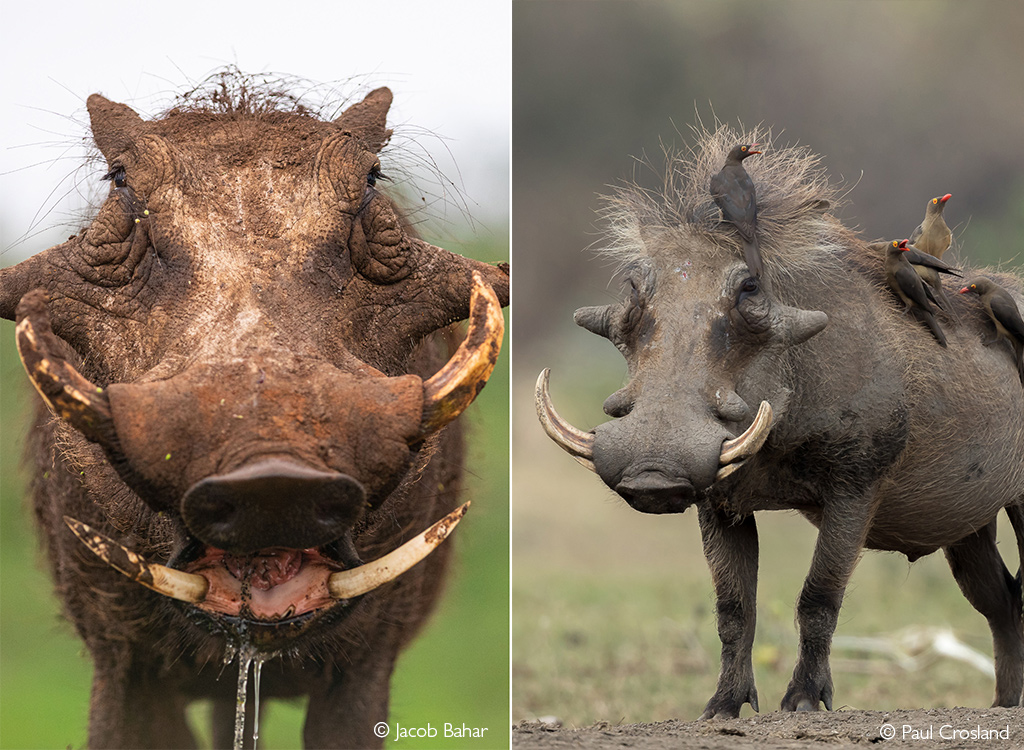The image is divided into two close-up pictures of common warthogs, separated by a thin white border. In the left photo, a warthog faces the camera, revealing a rugged appearance with a muddy brown coat. Prominently, it shows two sets of tusks: a larger upper pair and a smaller lower pair emerging from its open mouth, from which drool or mucus is dripping. Its black nose, pink tongue, and small ears add detail to its less-than-attractive face. The blurry background shows a green field under a white sky. The photograph includes a © symbol with the name Jacob Bar at the bottom.

The right photo presents a side view of another warthog, predominantly gray with less mud than the first. This warthog has a thicker mane of gray hair and is adorned with four small black birds with red eyes and beaks perched on its back and head. Its tusks, like those of the first warthog, are white and curved. The animal stands on dirt, and the image only shows its front part, including the legs and the birds. This photo is credited to Paul Crossland, indicated by a © symbol at the bottom.